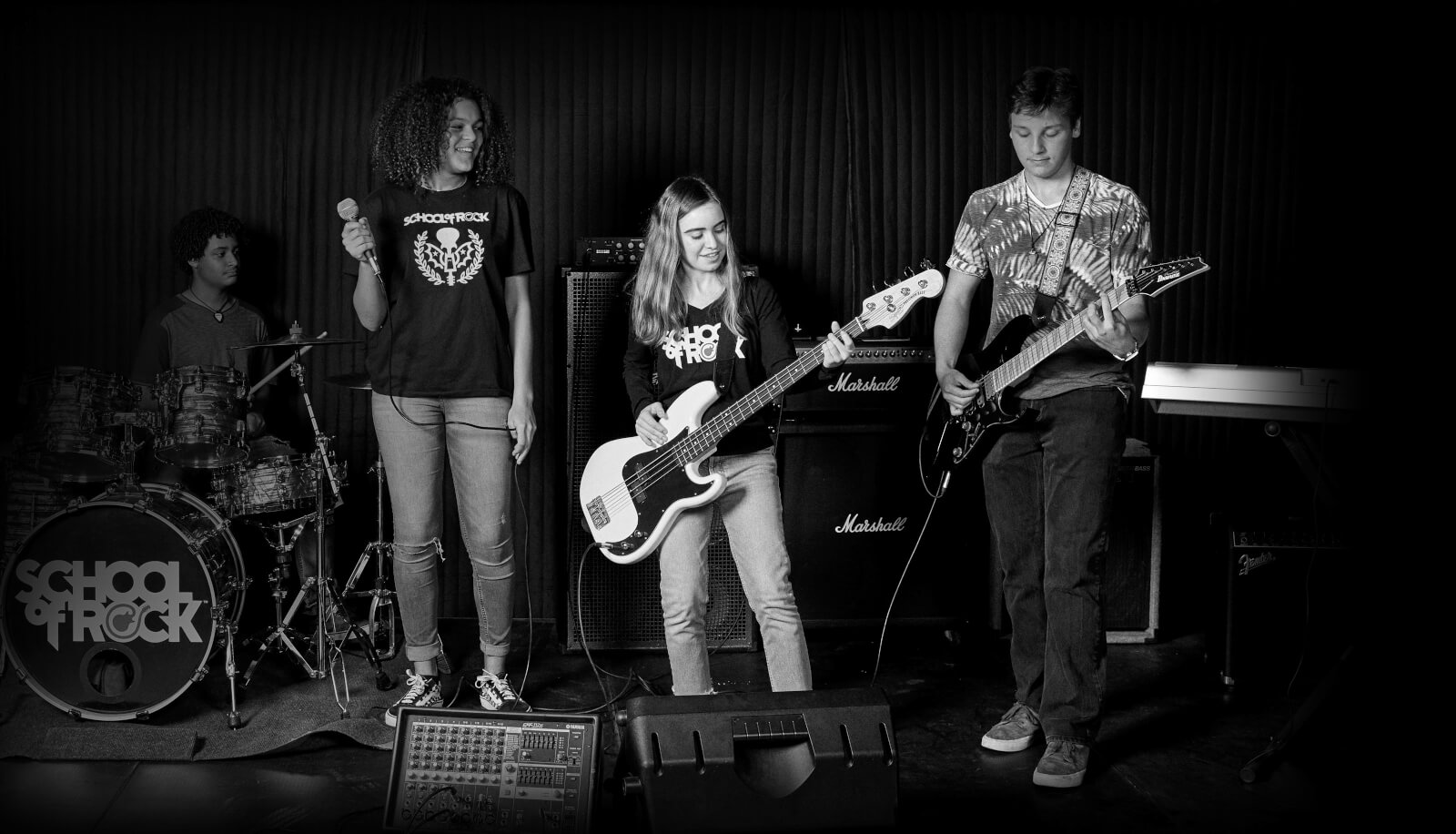This rectangular black and white photograph, wider than it is tall, captures a youthful band on stage under a dark backdrop. From left to right, there's a boy seated at a drum kit prominently labeled "School of Rock" in gray. Standing next to him is a tall young woman in a black School of Rock t-shirt and jeans, holding a microphone. To her right is a shorter girl with long blonde hair, clad in a similar School of Rock t-shirt, playing a white and black electric guitar. On the far right, another young man with a patterned or tie-dye t-shirt is looking down at his electric guitar, dressed in jeans and tennis shoes. Surrounding them are Marshall amps and other sound equipment, hinting at a live performance setting. The image evokes a concert-like atmosphere, with slight visibility of instruments and equipment adding depth to the scene.